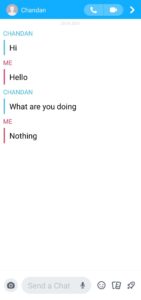This image is a cropped screenshot of a text message conversation, giving off a nostalgic vibe reminiscent of the early days of text messaging interfaces. The user interface features a simplistic design with a white background. At the top of the screen, you can see a user profile picture placeholder—a stock gray background with a white figure. To the right of the profile picture is the contact's name, "Shandon," with two buttons on the far right designated for phone and video calls.

Centered just below this header, the date of the conversation is displayed in a small gray font. The messaging interface begins with Shandon's name in blue, accompanied by a vertical blue line to the left of his message, which reads "hi." Immediately below, the user’s responses are denoted by "Me" in purple, with a corresponding vertical purple line to indicate their responses. The exchange proceeds with Shandon inquiring, "what are you doing?" followed by the user's curt reply, "nothing."

Each text message is color-coded by sender: blue for Shandon and purple for the user, with thin vertical bars to the side of each message reinforcing this color code.